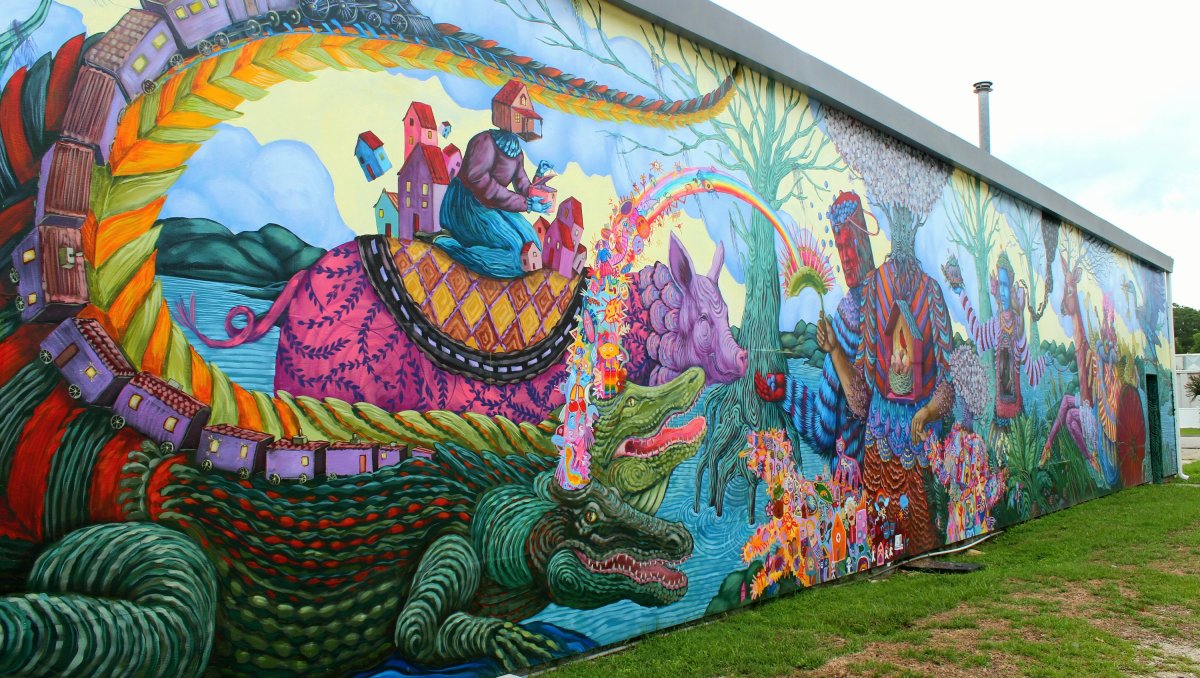The image features a stunning mural painted on the side of a concrete building surrounded by green and some patches of brown grass. The artwork is a vivid tapestry of various themes and colors, including blues, purples, reds, yellows, and greens. Dominating the left side of the mural is a green alligator with red stripes and an orange-green patterned pathway along its back. Atop the alligator, a purple train snakes through the artwork. Adjacent to the alligator is an enormous hybrid creature with a pig’s body, oversized and patterned like a cow, adorned with a yellow saddle bearing orange and yellow diamonds. Perched on this creature is a person dressed in a peculiar outfit with a house for a head, surrounded by small pink houses.

Further to the right, the mural depicts a sprawling tree with spiky limbs rooted in water. A rainbow arches above as various fantastical creatures and elements fill the space, including a blue-faced figure resembling the Tin Man holding a bird and a red-faced figure with blue and purple-lined fur, clutching blue marbles. A Tree-Man stands near the central tree, seamlessly blending human and tree elements. In the background, green mountains and another hybrid entity suggestive of a deer and bird are partially visible. The mural ends with a door on the far right next to a drain opening. This captivating, abstract piece serves as a testament to the limitless bounds of artistic expression.